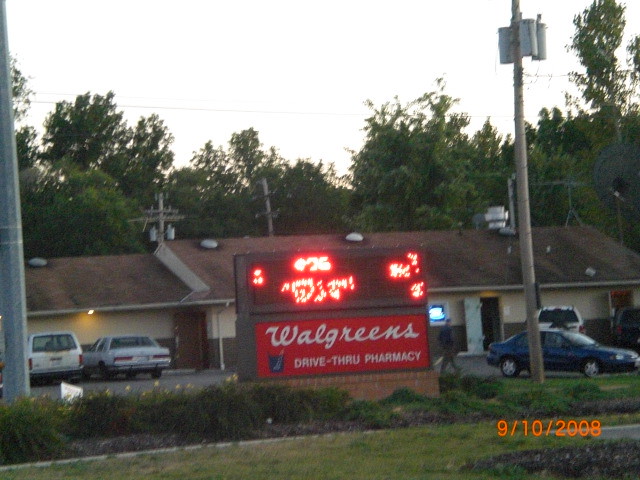In this photograph, the focal point is the exterior of a building, prominently featuring a malfunctioning Walgreens sign. The sign's upper panel is illuminated with red writing, but exhibits various blotches and lines indicating a technical glitch. Below this glitchy panel is the distinct Walgreens logo, written in a graceful cursive script in white. Accompanying the logo is a smaller descriptor stating "drive-through pharmacy."

Beyond the sign, a tan and brown building with a reddish-brown roof can be seen. This structure, which might either be the rear side of the Walgreens or a separate establishment like a motel, doesn’t quite match the typical Walgreen's appearance.

The parking lot in the foreground contains several vehicles, ranging from SUVs to sedans, in colors such as white, dark blue, gray, and tan. Adding a touch of nature to the scene, a flower bed is situated in front of the sign, adorned with what appears to be lilies or ornamental grasses. A sidewalk runs ahead of this floral arrangement, followed by a strip of green grass, creating a layered composition from the sidewalk to the sign, and then to the building in the background.